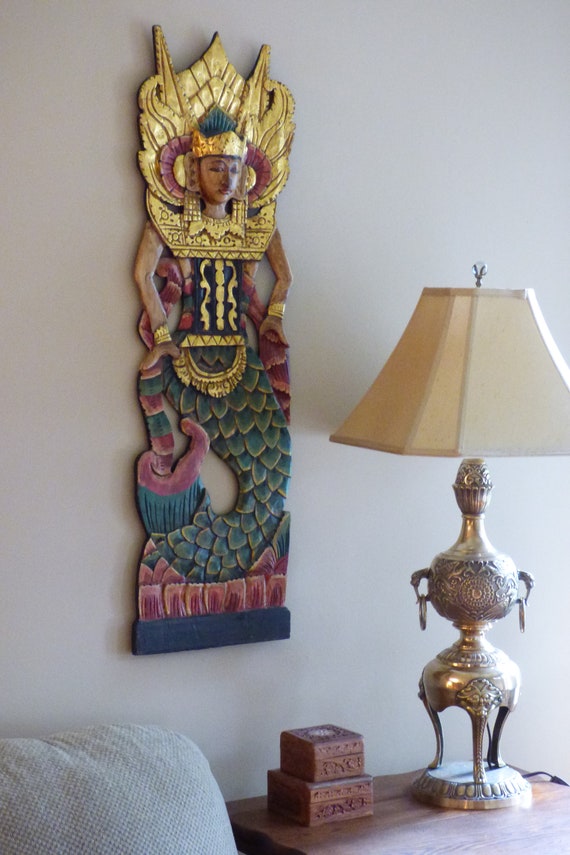This photograph captures a section of a tastefully decorated living room, prominently featuring a detailed handmade wooden plaque mounted on the light beige wall. The plaque, possibly of Southeast Asian origin – Indonesian or Thai, showcases an intricate carving of a serious-faced woman depicted as a mermaid. Her lower body, adorned with teal green scales and a gold-accented tail, conveys a sense of fluid movement. The mermaid is crowned with an elaborate gold headdress, which includes a central pointed element and dual pointed horns. A teal crest resembling a fin tops her crown, accompanied by pinkish-red horns extending from the sides of her ears. She wears ornate gold bracelets on her wrists, with her right hand positioned on her hip and her left hand delicately holding a richly decorated fabric scarf that wraps around her body and trails along the plaque's blue base. The carving includes graceful perforations around the arms and the undulating tail, enhancing its three-dimensional effect.

Adjacent to the plaque is a wooden end table, partially visible beside the edge of a beige-green sofa. The table holds two intricately carved wooden boxes, stacked one atop the other, which echo the cultural motifs of the plaque. A silver lamp with elaborate oriental carvings, topped with a regular fluted shade and glass finial, completes the decor, adding an elegant touch to the scene. The lamp’s design harmonizes with the artistic theme established by the wall plaque, making the whole setting a cohesive and culturally rich vignette.